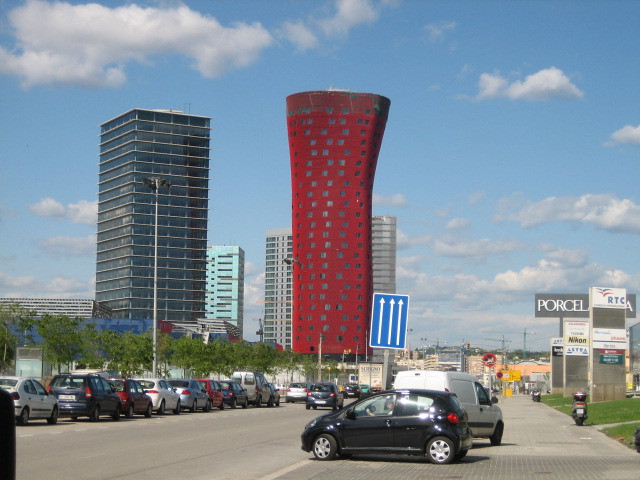This is a detailed image of a city street during daytime, captured in a vertical rectangular frame. In the foreground, several cars are traveling bumper to bumper away from the viewer, with a small two-door black hatchback prominently positioned as it appears to merge onto the road. Various vehicles of different colors, shapes, and sizes are also seen either parked or driving along the sidewalk.

To the right of the street, there are multiple vehicles coming in from a side road, blending into the flow of traffic. There are billboards, trash barrels, and small lights lining the sidewalk, and a mixture of green grass and shorter trees adding a touch of greenery to the scene.

The background features a cluster of tall buildings, including a distinctive, cylindrical red skyscraper with a curved top, a black cubic tower, a light teal building, and several typical gray concrete ones. The sky is vibrant blue, dotted with white and gray puffy clouds, lending a picturesque backdrop to this cityscape. The combination of photographic and somewhat artistic elements gives the image a unique and dynamic appearance.